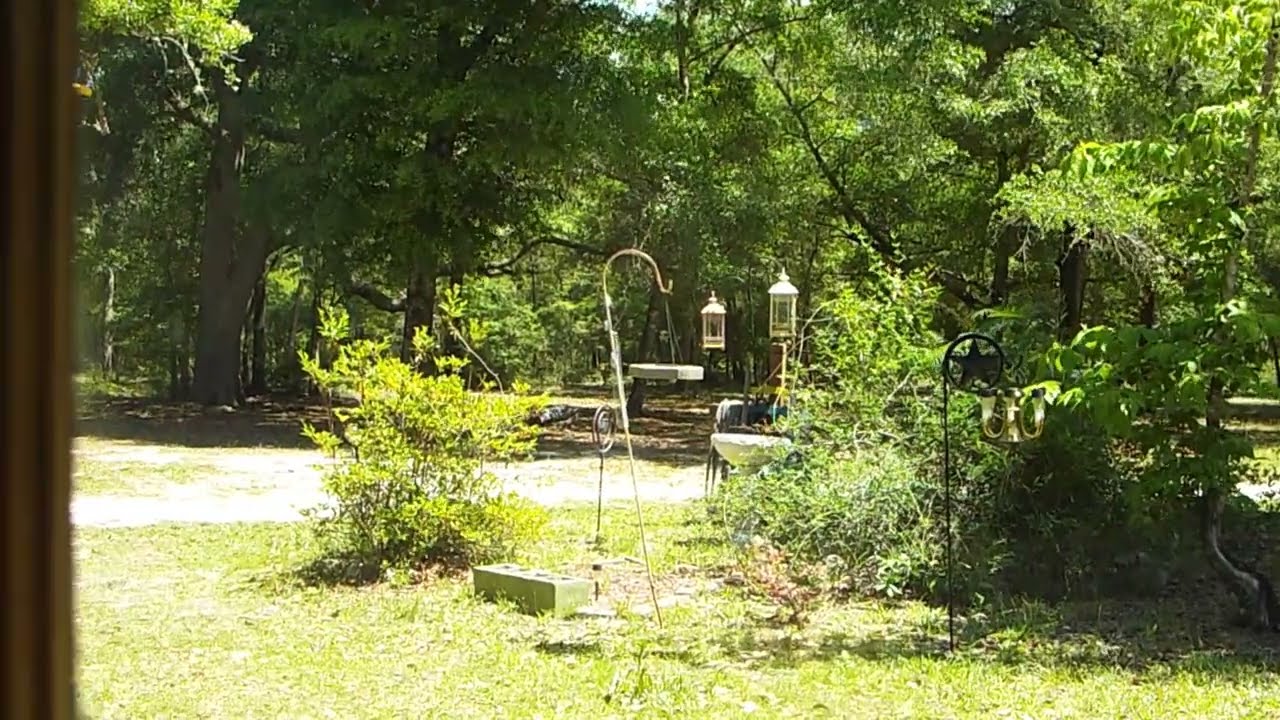The photograph captures a lush, green backyard on a sunny day, viewed from the inside through a window, evidenced by the window frame on the far left. Central to the image is a metal hanging bird feeder suspended from a chain on a long metal pole, with a cinder block on the ground nearby. Beyond the bird feeder, old-style gas candle lamps with glass windows line a path that runs horizontally across the midsection of the image, flanked by short grass that appears patchy in places. In the foreground, a concrete bird bath adorned with some greenery is present. The background reveals a dense woodland with large trees that cast shadows and obscure much of the sky, allowing only brief glimpses of blue through the thick canopy. The scene is imbued with the tranquility of a sunlit, tree-covered garden punctuated by various lawn ornaments and fixtures.